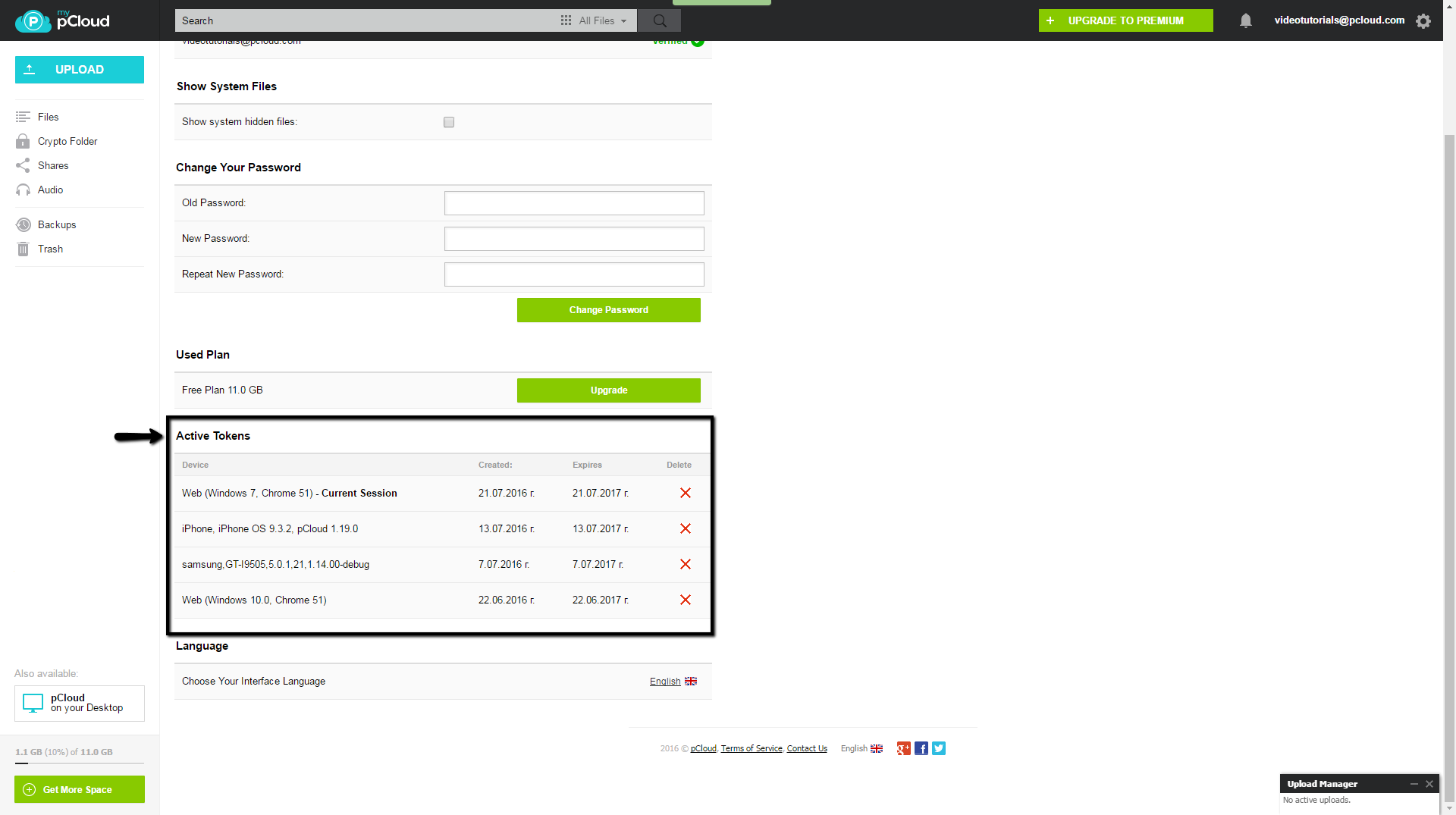This desktop screenshot captures the interface of a cloud storage website called "mypcloud." The logo, positioned at the top left, features a cloud icon with the letter "P," indicating a cloud computing or data storage service, which allows users to save data remotely rather than on their local devices.

On the left-hand side of the interface, a vertical menu presents various options: 
- **Upload** button for adding files.
- **Files** to view stored content.
- **Crypto Folder** for encrypted storage.
- **Shares** for sharing files with others.
- **Audio** for managing audio files.
- A separating line.
- **Backups** for system backups.
- **Trash** for deleted items.

At the bottom of this menu, there's a section promoting the availability of pCloud's desktop application, encouraging users to download it.

The main content area to the right of the menu displays details about the user's storage usage. At the top, it shows that 1.1 GB of the available 11.0 GB (10%) is being utilized. There's a button to purchase additional storage space.

Below this, the interface includes what seems to be a tutorial section featuring the "Active Tokens" functionality, encircled in a black square and highlighted with an arrow. Details displayed include:
- The current session on Windows 7 using Chrome 51.
- A list of other devices accessing the account, such as an iPhone, a Samsung device, and another session on Windows 10 with Chrome 51.

It also shows information such as the token creation date, expiration date, and options for token deletion.

The footer at the bottom of the page includes a copyright notice from 2016, indicating that the screenshot was taken in that year.